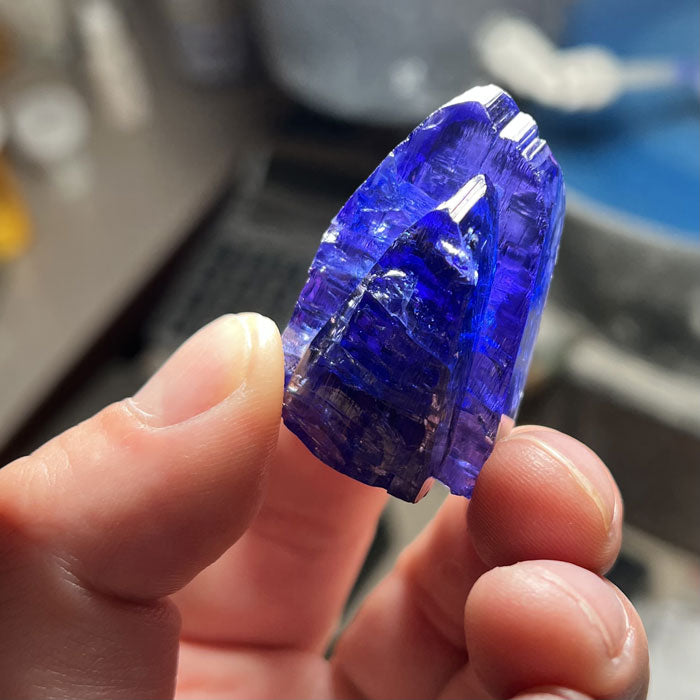The image is a close-up color photo of a man's hand holding a vibrant, deep blue crystal. The hand, with large fingers and short, unpainted nails, dominates the foreground, making the ridges of the fingerprints clearly visible. The crystal, held between the fingertips, exhibits a craggy, irregular shape with noticeable carving marks and round edges. It appears to be composed of two distinct sections: one is flat at the bottom and rises in an arched, jagged structure resembling an arrowhead, while the other section juts out like a triangular formation. The crystal is translucent, allowing light to pass through its lustrous surface, and it also reflects light, adding to its striking appearance. In the background, there is a blurry, indistinguishable scene with hints of blue and gray, possibly a desk and a calculator. The gem, despite some scratches, stands out as a beautifully detailed mineral specimen.